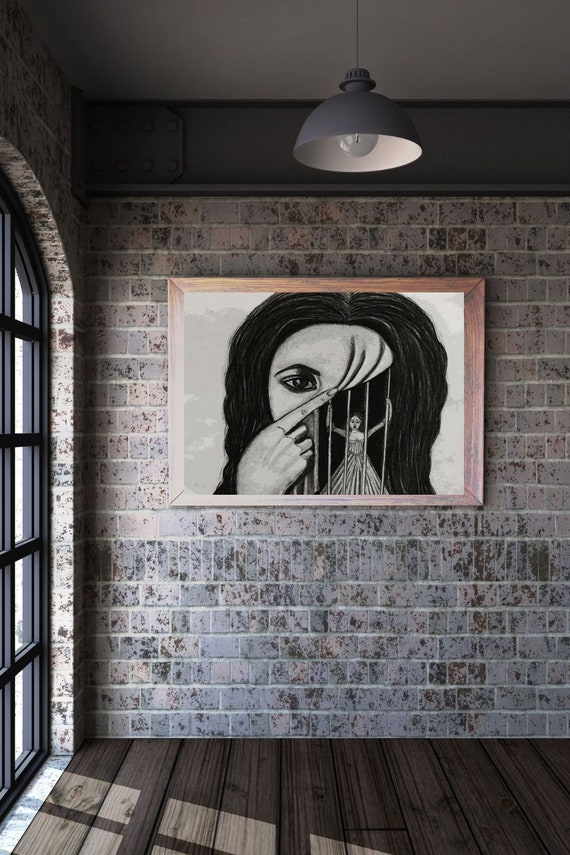The image features a detailed painting mounted on a brick wall, framed with a tan colored wood. The painting is prominently centered and depicts an abstract scene of a woman's face, her gaze directly engaging the viewer. She pulls her nose diagonally with her index finger, revealing another woman behind bars, creating the illusion that the jailed woman is inside her face. The distressed woman behind the bars wears a long, frilly dress with ruffled long sleeves and grips the bars with both hands. The outer woman has wavy black hair parted in the middle. The wall is a mix of brown and slightly red hues, adding a rustic feel to the setting. The wood floor beneath and a single light hanging from the ceiling illuminate the scene. To the left of the painting, light filters in through a window near an arched doorway, enhancing the ambiance.